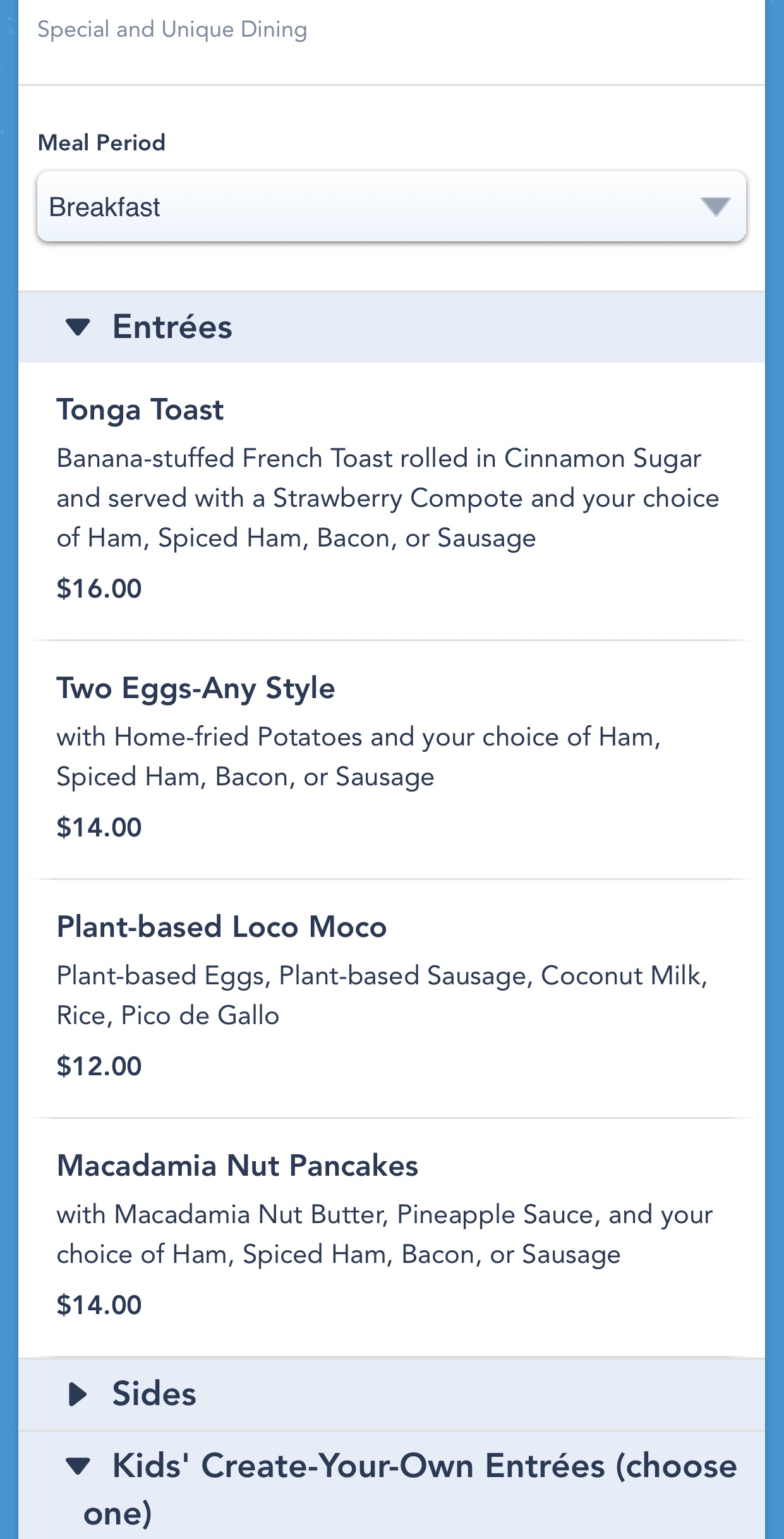The image showcases a menu with a blue-bordered background, providing a visually appealing dining experience. The menu details various breakfast options, each presented within a blue rectangle. 

Highlighted items include:

- **Tonga Toast**: Banana-stuffed French toast, rolled in cinnamon sugar, accompanied by strawberry compote, and a choice of ham, spiced ham, bacon, or sausage. Priced at $16.
  
- **Two Eggs Any Style**: Served with home-fried potatoes and a choice of ham, spiced ham, bacon, or sausage. Priced at $14.
  
- **Plant-Based Loco Moco**: Includes plant-based eggs, plant-based sausage, coconut milk rice, and pico de gallo. Priced at $12.
  
- **Macadamia Nut Pancakes**: Topped with macadamia nut butter and pineapple sauce, served with a choice of ham, spiced ham, bacon, or sausage. Priced at $14.

Additionally, the menu offers sides and a section for kids to create their own entrees, catering to various tastes and dietary preferences.